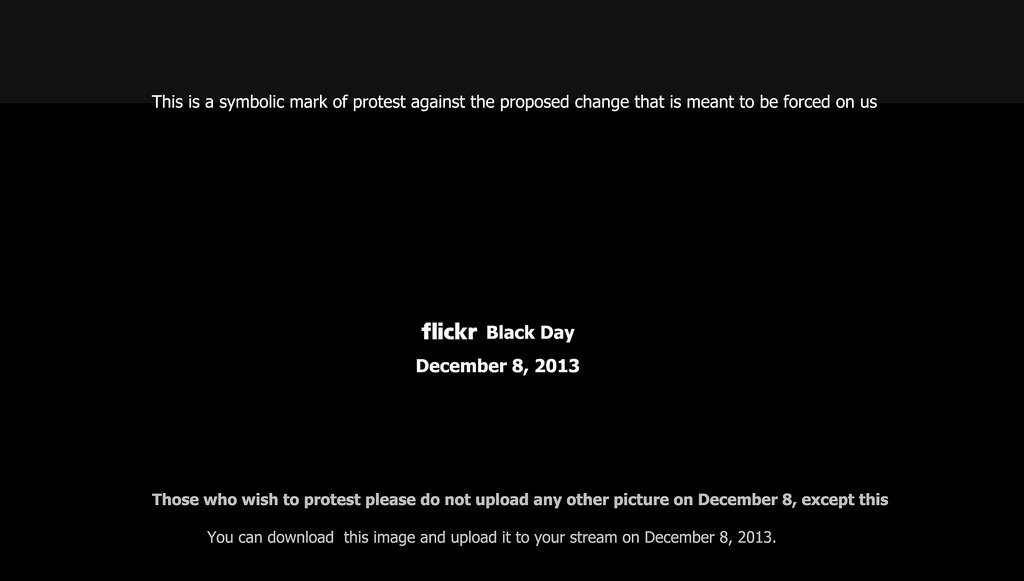The image is a black rectangle featuring white text. At the top, a sentence reads, "This is a symbolic mark of protest against the proposed change that is meant to be forced on us." Centered in the middle, two lines of text declare, "Flickr Black Day, December 8th, 2013." At the bottom, also center-justified, it instructs, "Those who wish to protest, please do not upload any other picture on December 8th except this. You can download this image and upload it to your stream on December 8th, 2013." The entire text appears white against the black background, with a subtle, slightly brighter gray band running horizontally across the top.